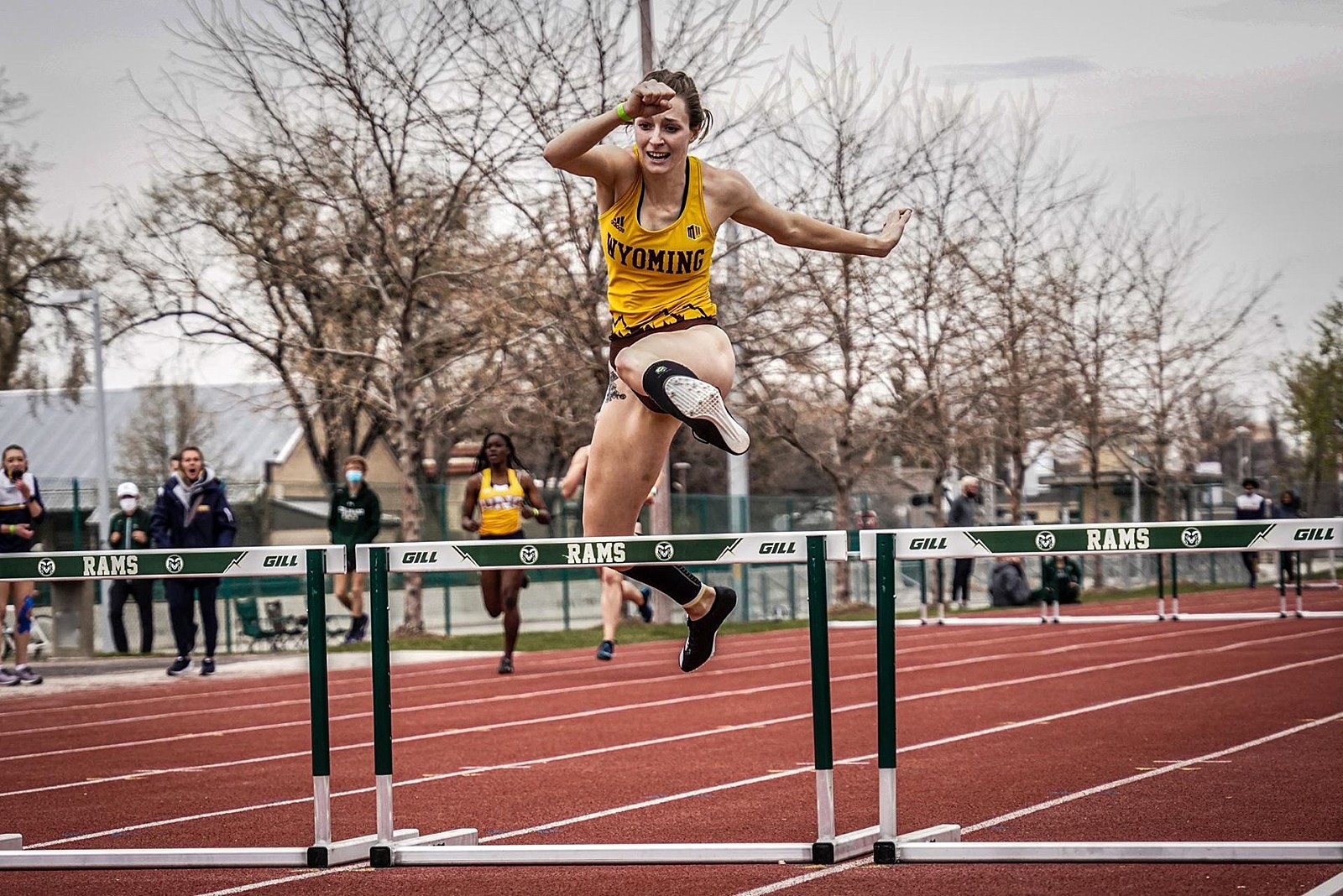The image depicts a dynamic moment during a relay race, capturing a college-aged woman mid-jump over a hurdle on a maroonish-brown track marked with white lane lines. The athlete, wearing a yellow tank top with "Wyoming" written in black letters and an Adidas logo in the top left corner, is in full stride, her muscular legs propelling her above the hurdle while her brown hair is neatly pulled back. She sports short black shorts and black shoes. The hurdle she leaps over has a white metal top part with "Rams" and "Gill" inscribed on it in black. Her face is a picture of intense focus, with her arms extended for balance. In the background, other runners, significantly behind her, strive to catch up. Spectators, some with masks on, cheer them on from the sidelines under a gray sky with bare trees and a few scattered leaves visible at the edges of the frame.